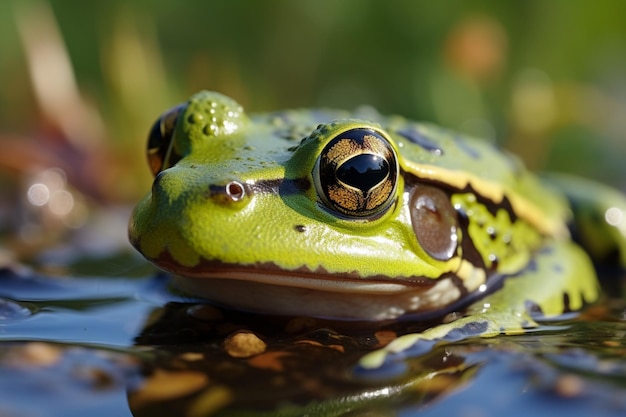This is a close-up, color photograph of a frog's face and part of its body, taken outdoors in a natural setting during the day. The background is blurred, displaying a mix of green, white, orange, and yellow hues, suggestive of an open field and a small, muddy body of water. The frog, predominantly bright green with dark, muddy streaks and black spots, is partially submerged in water. Its large eyes are black with a golden-yellow surrounding color, and there is a noticeable round brown spot behind its left eye. The underside of its mouth is an off-white or beige color, and its closed mouth features a yellow line on the side of its body. The frog's eyelids are bumpy and round, adding to the texture and detail of its vivid appearance.